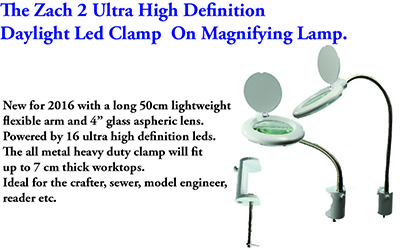The image displays the Zac2 Ultra High Definition Daylight LED Clamp-on Magnifying Lamp, a cutting-edge product introduced in 2016. This lamp features a robust 50cm lightweight, flexible arm that maneuvers effortlessly to your desired position and a 4-inch glass aspheric lens designed for precision work. It is powered by 16 Ultra High Definition LEDs, ensuring optimal illumination for tasks requiring meticulous attention to detail. The heavy-duty, all-metal clamp can securely attach to worktops up to 7cm thick, making it an ideal companion for crafters, sewers, model engineers, and avid readers.

To the right of the main image are three detailed pictures of this versatile device. One image highlights the sturdy clamp mechanism with its white clamping area and adjustable metal rod. The other two images showcase varying perspectives of the magnifying lamp, emphasizing the LED light source and the highly flexible arm, reminiscent of a hose lead, that provides versatile movement and positioning. At the end of the flexible arm, there is a circular magnifying lens encircled by a bright LED ring, designed to provide unparalleled clarity and brightness for any detailed task.